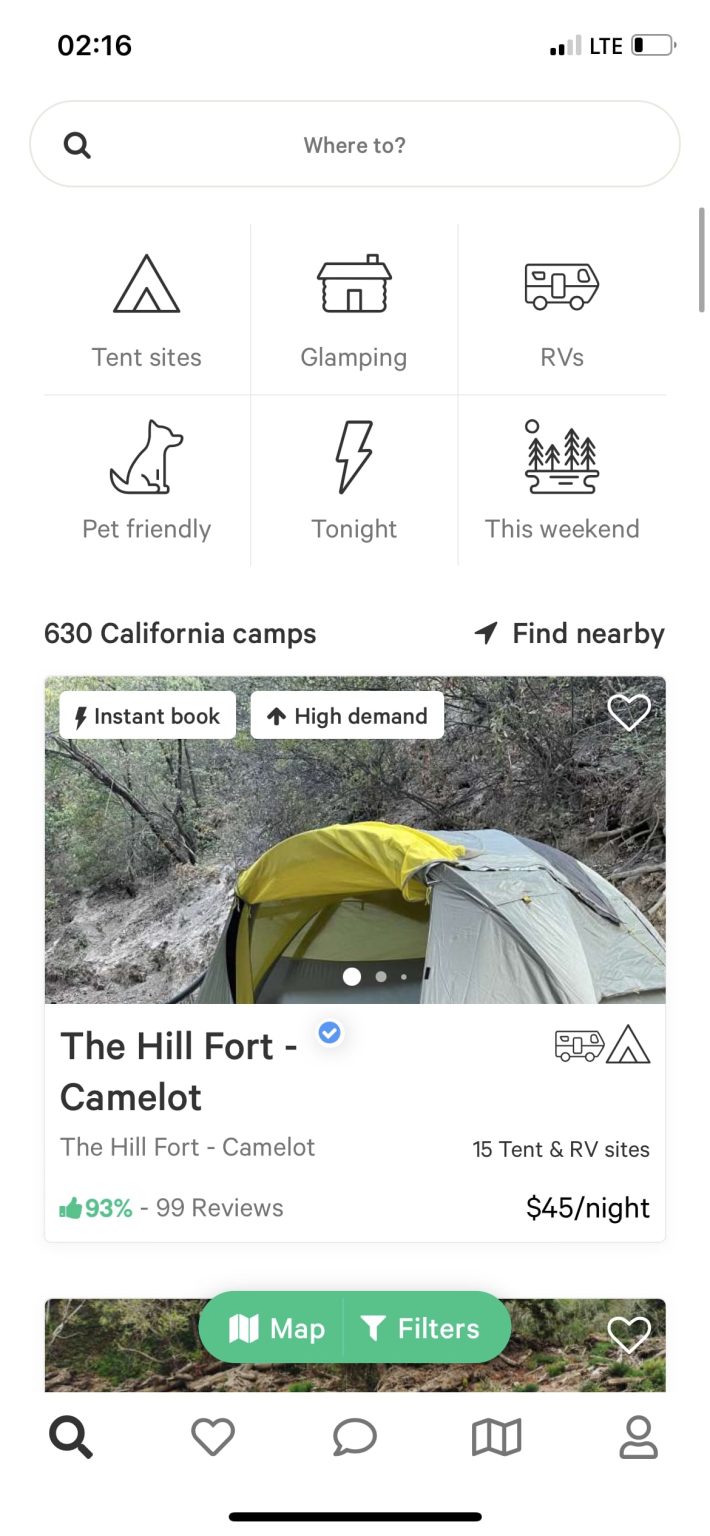This image displays a review site for a campsite. At the top of the screen, the time is shown as 2:16. Beneath that sits a "Where to?" search prompt. Below, six categories are organized in a 3x2 grid, each represented by a distinct symbol: "Campsites" features a pair of triangles, "Glamping" is denoted by a log cabin, "RVs" displays a picture of an RV, "Pet-Friendly" is illustrated with a dog icon, "Tonight" is marked by a lightning bolt, and "This Weekend" showcases an image of a lake flanked by trees. These visual symbols function as intuitive guides for the user.

Further down, the header announces "633 California Camps," accompanied by a photograph of a greenish-gray tent with a yellow interior, set up in a sandy area dotted with vegetation. Below the photo, the campsite is identified as "Hill Fort Camelot," which offers 15 tent and RV sites. The site boasts a 93% approval rating based on 99 reviews and is priced at $45 per night. Underneath this information, options are provided to view a map or apply filters for more refined searches.